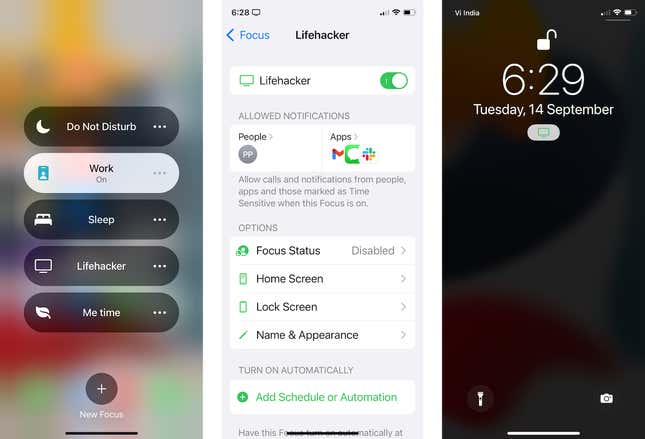The image showcases three distinct screens. The leftmost screen, which has a gray background, features several capsule-shaped icons in black. These icons represent different modes: the first one shows a moon symbol and is labeled "Do Not Disturb," while the second icon is for "Work." The "Work" mode is currently active, indicated by its gray highlight. Additionally, there are modes labeled "Sleep," "Lifehacker," and "Me Time," with the "Lifehacker" mode partially pulled up.

The rightmost screen appears to be the main interface of a device, displaying the date "September 14, 6:29 PM" at the top. This screen details the settings for the "Lifehacker" mode, which is highlighted in green because it is turned on. It shows options for allowed notifications, specifying certain people and apps that can bypass the "Lifehacker" mode settings for calls and notifications.